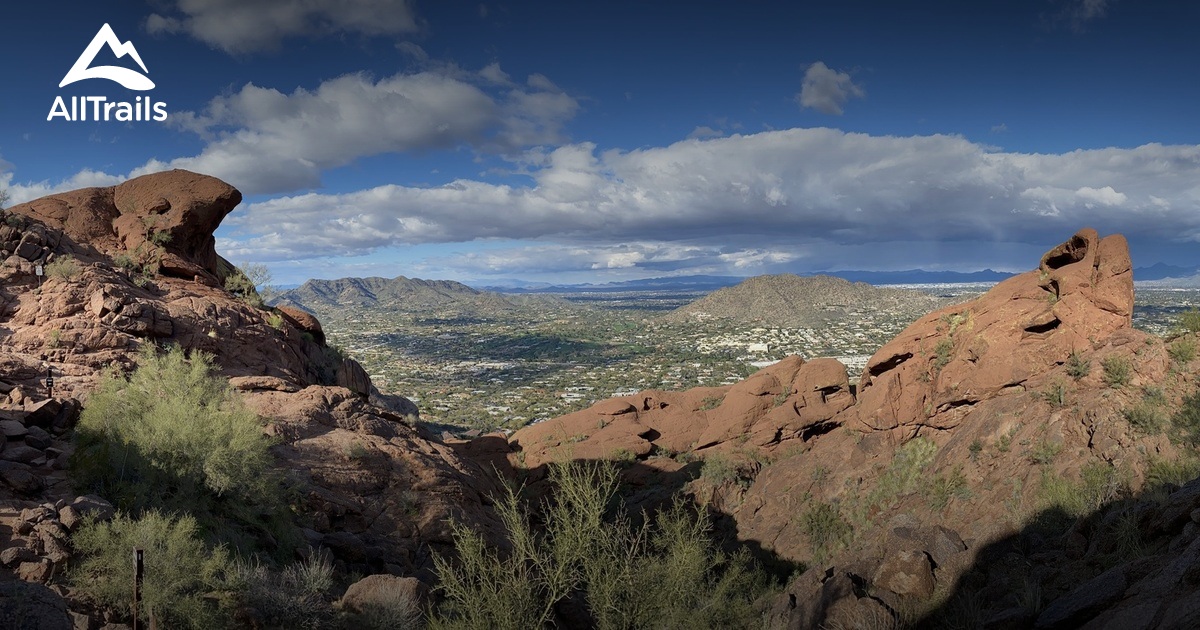This panoramic photograph features a rugged, mountainous outdoor landscape, adorned with the All Trails logo in the top left corner, indicating a prime hiking location. The sky, occupying the top half of the image, is painted in a vivid shade of blue with heavy, billowing thunderclouds beginning to gather and cast impending shadows over the scene below. The foreground is dominated by rough, reddish-brown clay and rock formations, interspersed with sparse green brush, suggesting challenging but walkable terrain, typical of regions like Utah, Arizona, or New Mexico. The land stretches out into a vast open valley and further into a series of distant mountain ranges, revealing layers of dirt brown, yellow, red, and orange hues. The rugged appearance of the landscape is accentuated by sharp, bumpy rock surfaces and patches of grass and sand. In the far distance, under the vast expanse of the "big sky," the horizon culminates in high, towering peaks, hinting at the extensive altitude and expansive views hikers might enjoy in this strikingly desolate yet beautiful terrain.